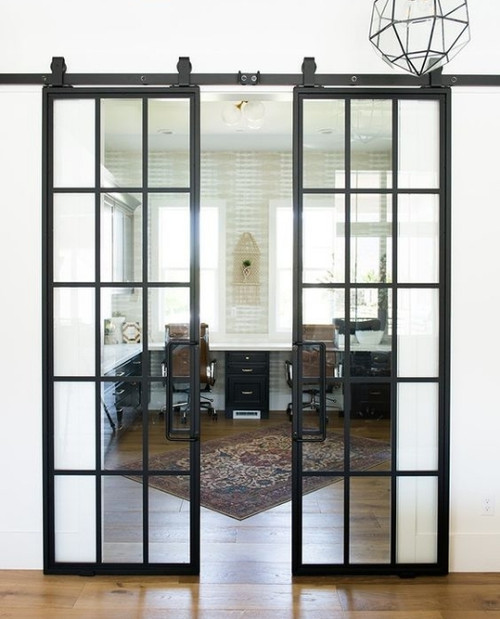This vertically aligned rectangular picture captures a glimpse into a home office through partially open sliding glass doors with dark brown metal frames. Each door features 15 rectangular panes of glass, organized in three columns and five rows. The doors slide along a dark brown metal bar situated at the top. The floor, covered in medium brown wood tiles with dark knots, extends into the adjacent room. The office space within is furnished with an L-shaped white desk, complemented by black drawers and a pair of rolling office chairs. Positioned at a diagonal on the floor is an area rug decorated in brown and gold patterns. Also present under the desk are file cabinets, and natural light streams in from two large windows positioned on either side of the desk, enhancing the room's bright and airy atmosphere. The color palette includes beige, white, brown, walnut, and black, creating a cohesive and professional work environment.